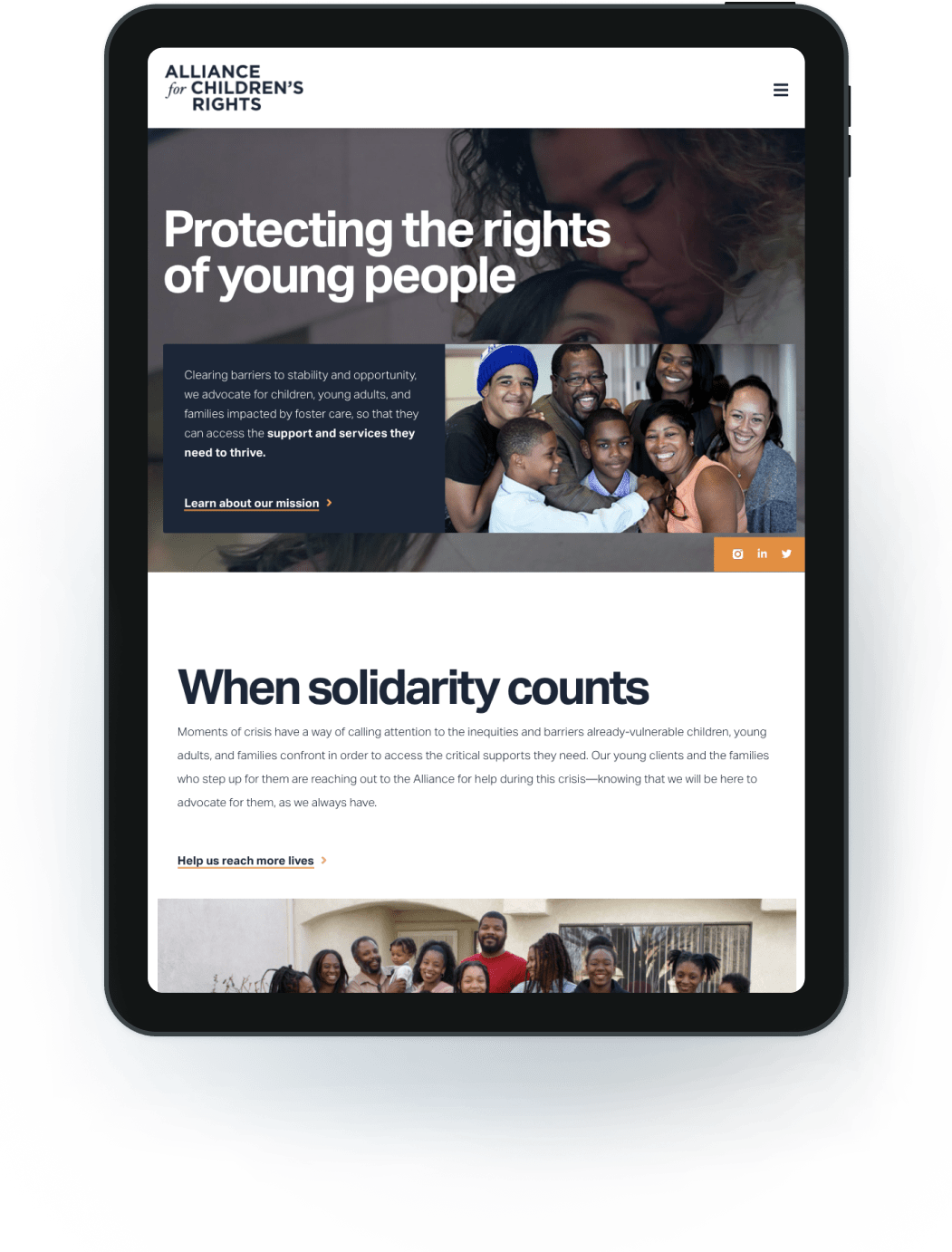This image captures an artistic rendering designed to resemble a tablet interface. The tablet features a distinct, thick black border. Prominently placed at the top is a rectangular white bar. On the left side of this bar, bold black lettering reads "Alliance for Children's Rights," while the upper right corner contains three stacked horizontal lines, suggestive of a menu icon. 

Beneath this white section is a semi-transparent banner image that sets the background for the main content. The banner displays a tender moment of a mother holding a child close to her chest, her head lowered as she kisses the child’s forehead. Superimposed on this background are the words "Protecting the Rights of Young People" in white lettering, partially blending into the image.

Dominating the lower portion of the banner is a clearly visible rectangular picture. On the right side of this rectangle is a photo of seven individuals, comprising two men, two young boys, and three women, suggesting they might be from a South American country. 

To the left of this photo, text in white reads: "Clearing Barriers to Stability and Opportunity. We advocate for children, young adults, and families impacted by foster care so that they can access the support and services they need to thrive." The phrase "support and services they need to thrive" is highlighted in bold white text. An orange underline emphasizes the bold white text "Learn About Our Mission."

In the bottom right corner, a rectangular orange button features white icons for Instagram, Indeed, and Twitter. Below in the white section, bold black text declares "When Solidarity Counts." 

In the bottom left corner, text reads "Help Us Reach More Lives," underlined in orange with a right-facing orange arrow next to it. The very bottom of the image appears to be the cropped top of a rectangular photo. This glimpse shows about ten people standing in front of a white building, all smiling warmly.

This detailed composition effectively communicates the organization’s mission to support and advocate for those affected by foster care.